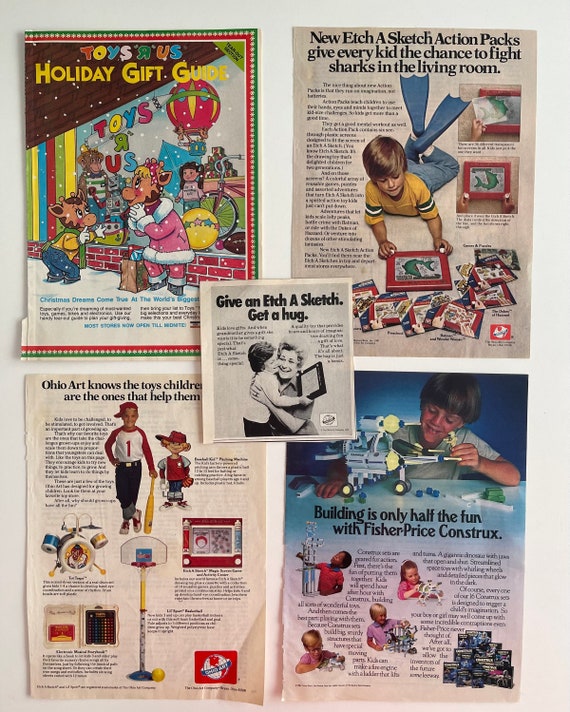This image contains five magazine advertisements arranged in a two-by-two grid with a smaller ad in the center, set against a white background.

1. **Top Left (Toys R Us Holiday Gift Guide)**: This colorful advertisement is bordered with festive red, white, and green decorations and showcases Toys R Us giraffes, Jeffrey and his mother, standing in the snow outside a store. The mother giraffe wears a pink and white coat, while Jeffrey wears blue jeans. Behind them is a red-bricked Toys R Us store adorned with images of a large monkey, a little girl, and a bicycle. The text reads, "Toys R Us Holiday Gift Guide," followed by, "Christmas dreams come true at the world’s biggest..." (cut off).

2. **Top Right (Etch-A-Sketch Action Packs)**: Set against a grayish-pink background, this ad features a young boy lying on his stomach, wearing a yellow T-shirt, jeans, and blue swim fins. He is drawing a green shark on an Etch-A-Sketch. The headline reads, "New Etch-A-Sketch Action Packs Give Every Kid the Chance to Fight Sharks in the Living Room," and includes additional images of Etch-A-Sketch creations.

3. **Bottom Left (Ohio Art)**: This page shows a young boy in a red baseball cap, red and white baseball shirt, and blue jeans standing next to a cartoon version of himself, similarly dressed. The partially visible text reads, "Ohio Art Knows the Toys, Children...Are the Ones That Help Them." Objects including a basketball hoop, a toy drum set, and various indistinct toys are also pictured.

4. **Bottom Right (Fisher-Price Constructs)**: This ad highlights a boy playing with a spaceship-like model made from Fisher-Price constructs. The headline states, "Building is only half the fun with Fisher-Price Constructs," supplemented with images of other children playing with similar construct toys.

5. **Center (Etch-A-Sketch Hug)**: The black-and-white ad in the center features a nostalgic scene of a small boy hugging an older woman, accompanied by an Etch-A-Sketch. The simple yet evocative text reads, "Give an Etch-A-Sketch, Get a Hug."

This detailed composite draws on recurring elements from each description, emphasizing shared observations and details to create a comprehensive caption.